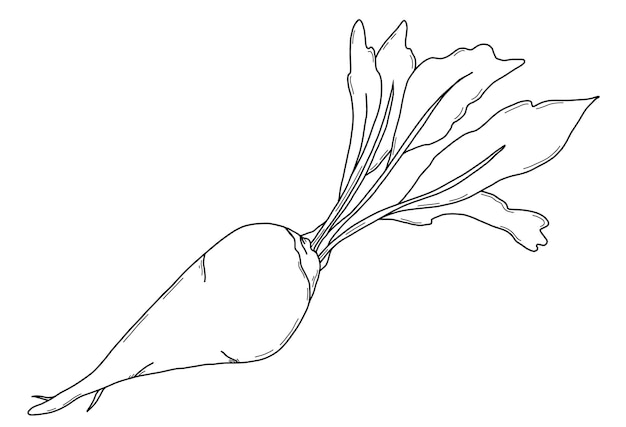This is a black and white thin line sketch of a turnip. The vegetable is depicted in pen and ink with a minimalistic approach, featuring very thin lines and sparse detailing. The turnip, oriented towards the left, exhibits two small roots at its pointed tip and features a subtle definition at its base. Emerging from the upper right side are five small leaves on longer stems, with minimal redundant lines to suggest volume. The entire illustration, uncolored and devoid of labels or signatures, is set against a white background, capturing the essence of a gardening book diagram or a cooking site icon.